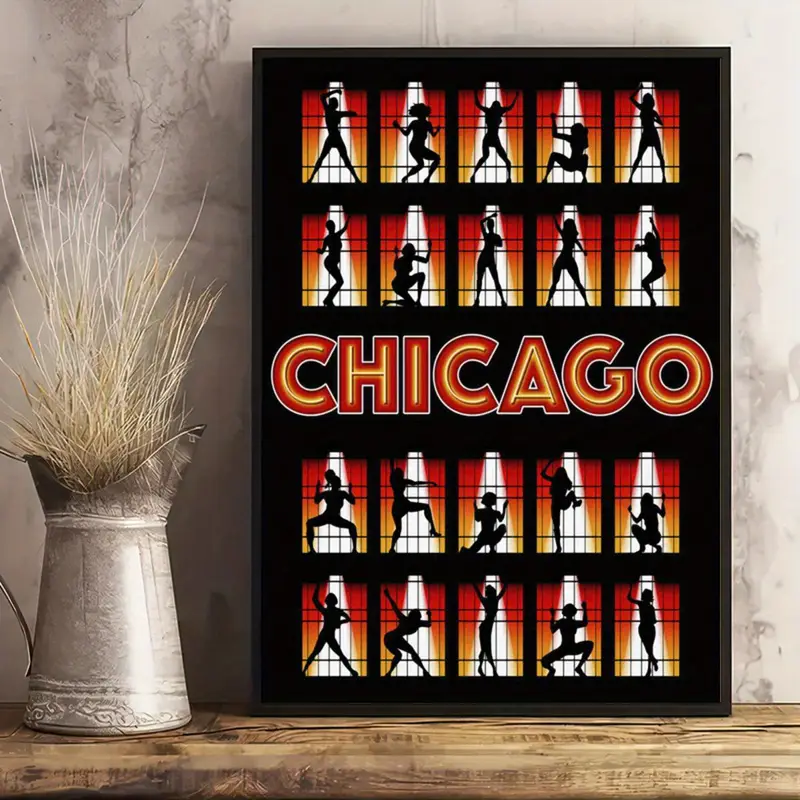The image depicts a detailed poster for the musical "Chicago" placed on a wooden shelf with a gray marble-like background. The poster, framed in black, prominently features "Chicago" in large yellow bubble letters on a red background with a white border at the center. Surrounding the central text are images of female dancers arranged in four rows and five columns. Each image has an ombre effect, transitioning from red at the top to orange in the middle and yellow at the bottom. The dancers are silhouetted in black, each striking different dance poses under white triangular spotlights. On the left side of the shelf, there is a silver water pitcher with what looks like decorative yellow and brown plants resembling tumbleweeds emerging from it.